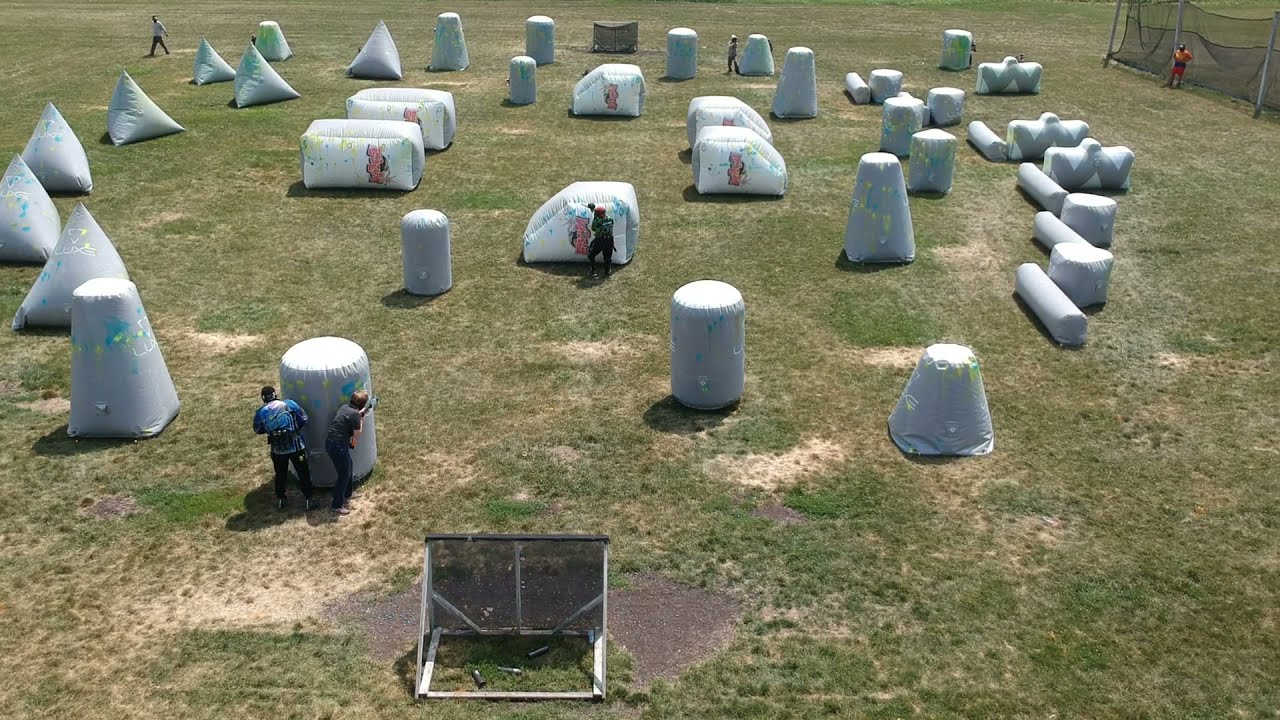The image depicts a vibrant paintball arena, possibly captured from an aerial perspective. The arena is strewn with a variety of inflated covers, including pyramids, ovals resembling punching bags, rectangles, and some irregular shapes. These obstacles are predominantly grey and white, marked with paint splatters and graffiti-like designs. Two players are visible in the bottom left corner, with one wearing a blue shirt peeking out from the left side of a punching bag-shaped cover, and the other in a grey t-shirt and jeans looking out from the right side. A man in the middle, dressed in a green shirt, red helmet, black cargo pants, and black shoes, is also seen behind a cover, scanning the upper part of the arena. In the background, a net attached to posts can be observed in the top right corner, behind which stands a person wearing short red pants, an orange shirt, and a cap, potentially serving as a referee. The field, resembling a soccer pitch, is filled with these temporary obstacles arranged mostly in a circular pattern, creating a dynamic and chaotic battleground for the players.